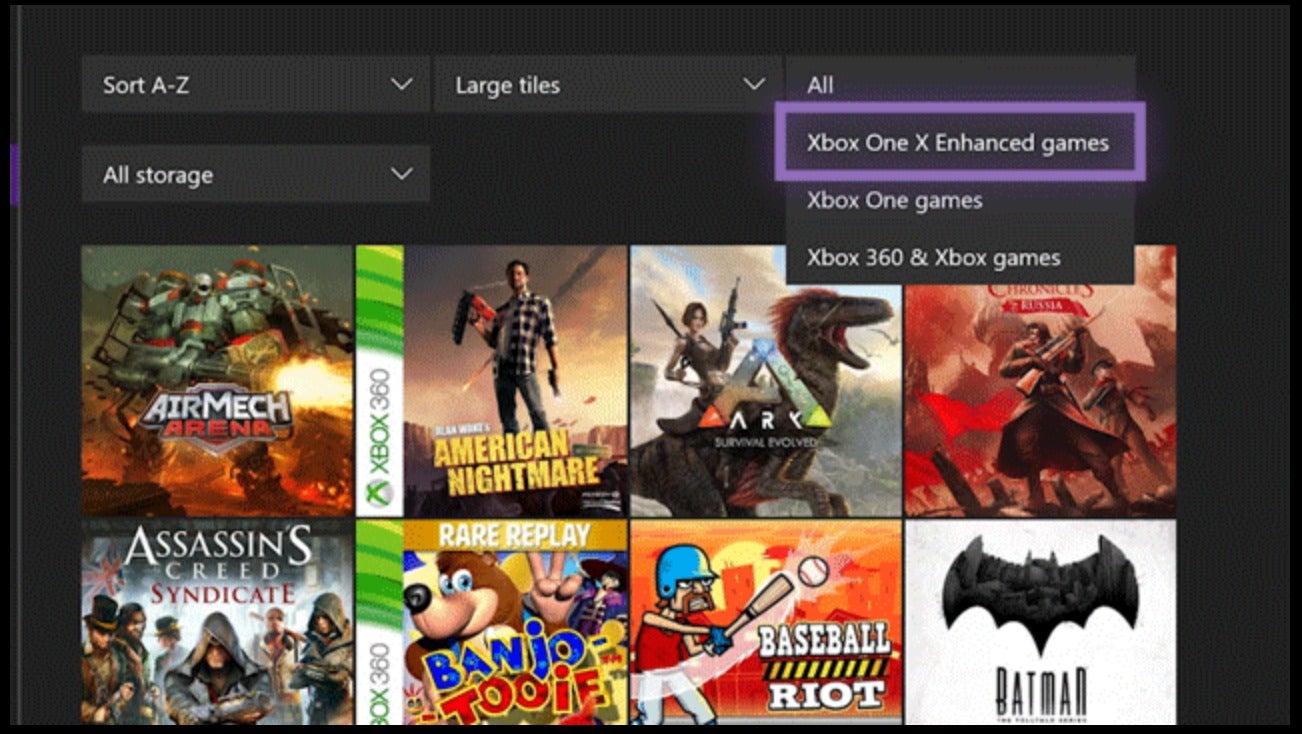The image showcases a user interface for an Xbox gaming library. At the top, there is no specific label, but four prominent drop-down boxes are presented, offering options for sorting and filtering the visible content. The drop-down boxes include the sorting options from A to Z, a filter for all storage options, another for displaying large tiles, and a comprehensive filter labeled “All.”

One of these drop-down menus has been expanded, revealing options for filtering the library by game category: "Xbox One Enhanced Games," "Xbox One Games," "Xbox 360," and "Xbox Games." There are eight visible game thumbnails displayed beneath these menus, each representing a different game title available to play. The thumbnails shown include "Assassin's Creed Syndicate," "Baseball Riot," "Batman," "Banjo-Tooie," "American Nightmare," "ARK," "Air Mech Arena," and "ARK Chronicles." Due to the expanded drop-down menu, part of the screen is obscured, making it difficult to view the first word of the game's titles.

The interface has a sleek, black background, and the game icons are displayed in a large, easily visible format. The active selection within the drop-down menu is outlined with a purple border, indicating the current focus, which changes as the user navigates through the list. This navigation likely involves using a mouse to hover over and select the desired category, with the purple border shifting accordingly.